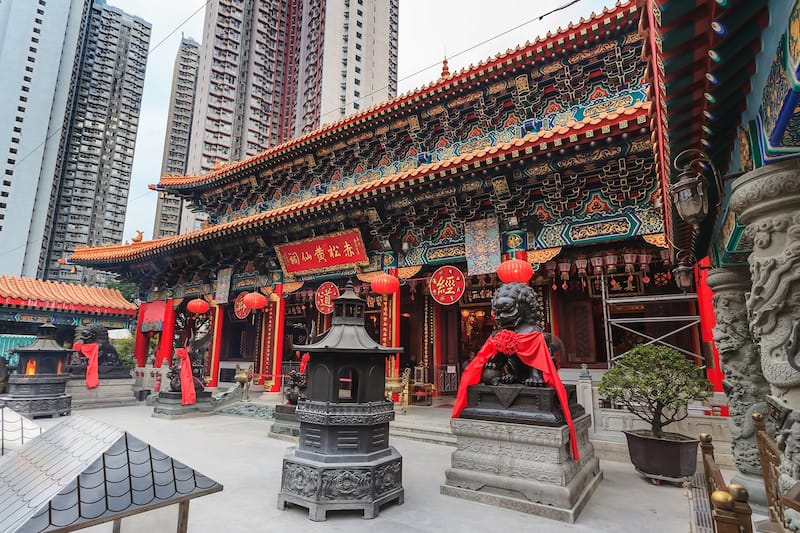The photograph captures a Chinese temple characterized by its intricate and ornate architecture. The temple, showcasing a striking combination of black with yellow or gold accents, features prominent red pillars and traditional Chinese signage. Flanked at the temple’s entrance are two sculpted lion statues draped with red cloth over their necks and shoulders. These statues guard a small concrete courtyard that includes planters with bonsai trees and other minimal greenery. In the background, modern high-rise apartment buildings tower over the scene, juxtaposing the ancient elegance of the temple with contemporary urban elements. The sky above is a muted light gray, further highlighting the vibrant red and gold details of the temple's design.